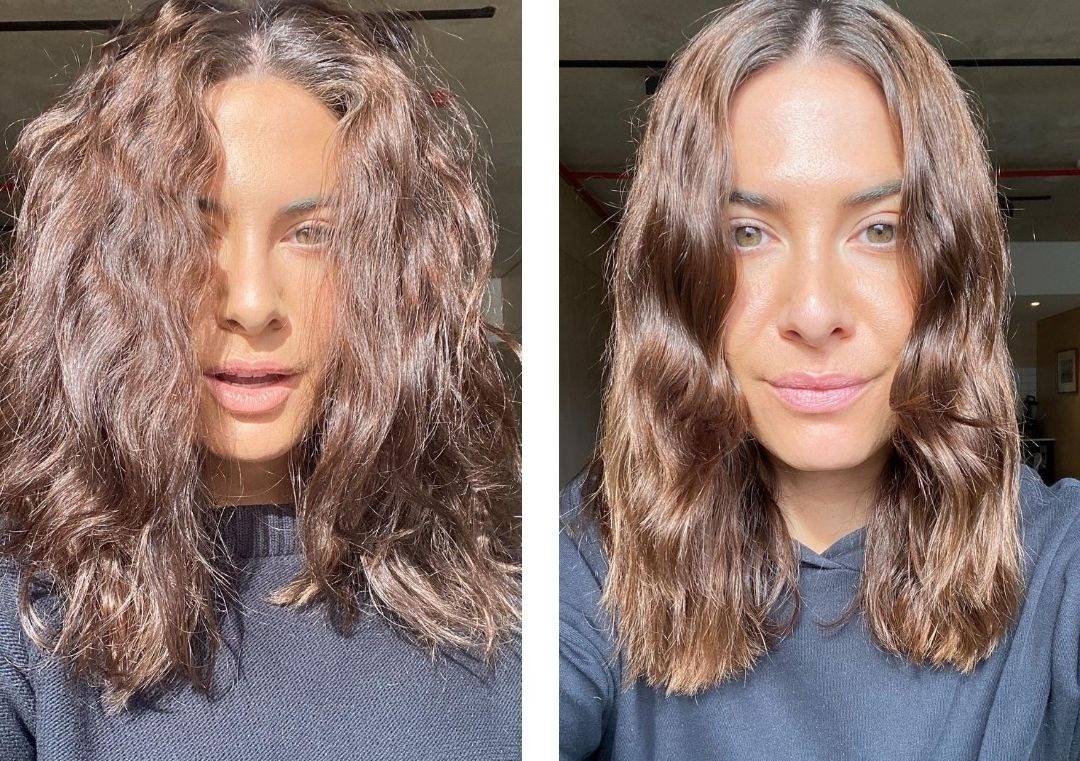The photograph is a side-by-side comparison capturing a before-and-after transformation of a young woman's hair. In both close-up selfies, the woman, who has long brown hair, is wearing a dark grey top and is looking directly at the camera. In the left image, her hair appears super frizzy, unwieldy, and unmanageable, giving it a fluffy appearance as if she has been shaking it out. Her mouth is slightly open, and she is not smiling. In contrast, the right image showcases her hair as significantly more tame, flat, and well-combed, though it retains some waviness and falls a couple of inches past her shoulders. Here, she appears more put together, with a noticeable smile on her face, potentially indicating increased confidence or satisfaction with her appearance. The lighting in both images suggests she is standing near a window or garage door, as her hair is shining in the sun.